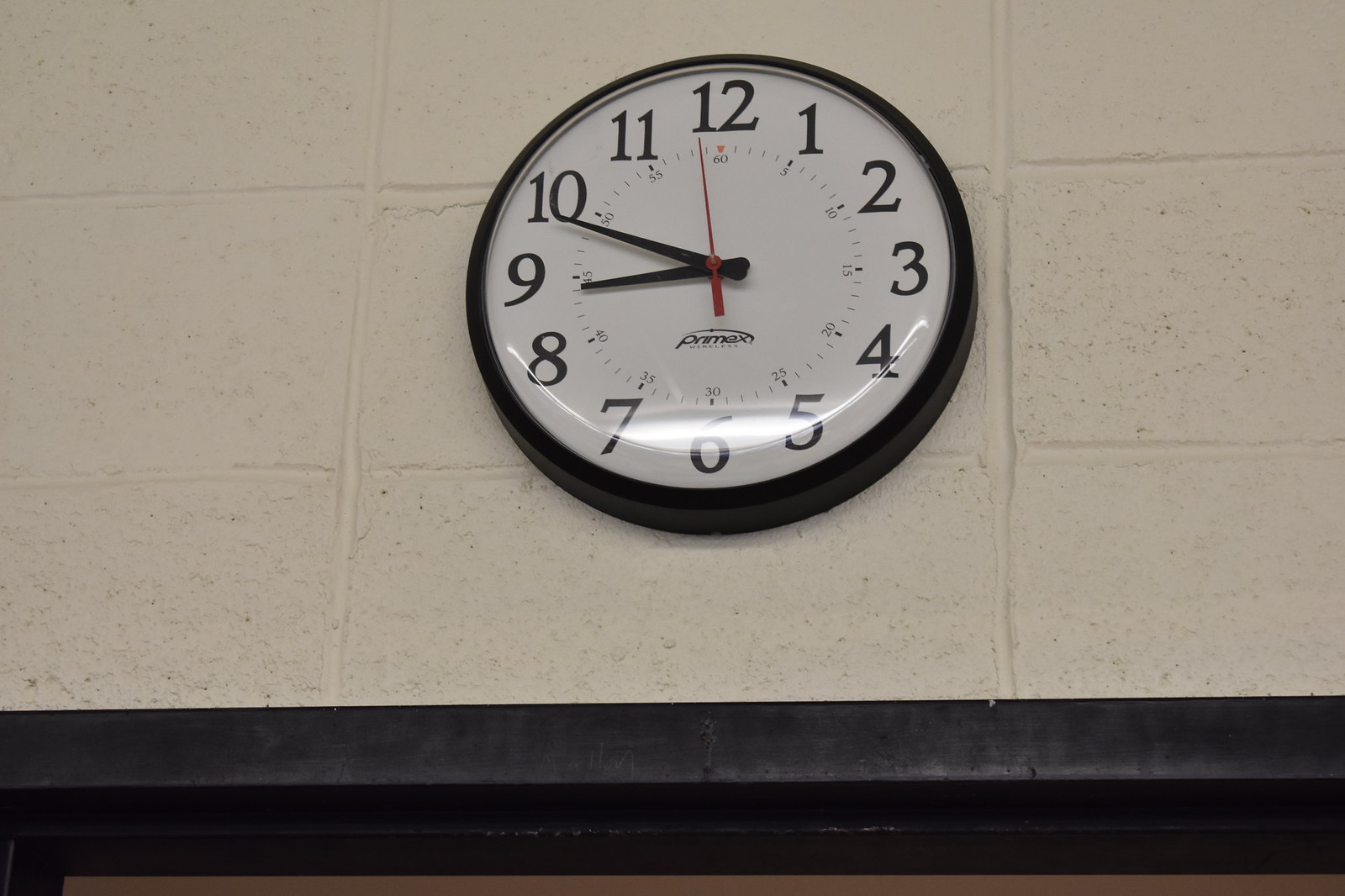The photograph showcases a circular clock mounted on a white brick wall. The clock features a black plastic border encircling its face. The clock face is white with bold black numbers from 1 to 12 denoting the hours. Each number is positioned around the dial. In the center, the clock hands are visible—two long black hands indicating the hour and minute, and one slender red hand for the seconds. The brand name "Primex" is inscribed in black text in the middle of the face, just below the clock hands. Surrounding the central hands are smaller numerical indicators from 60 back to 0, identifying the seconds or minutes. The time displayed is approximately 8:50. The clock is affixed to a wall constructed of large, rectangular white stone blocks with a textured, bumpy surface.